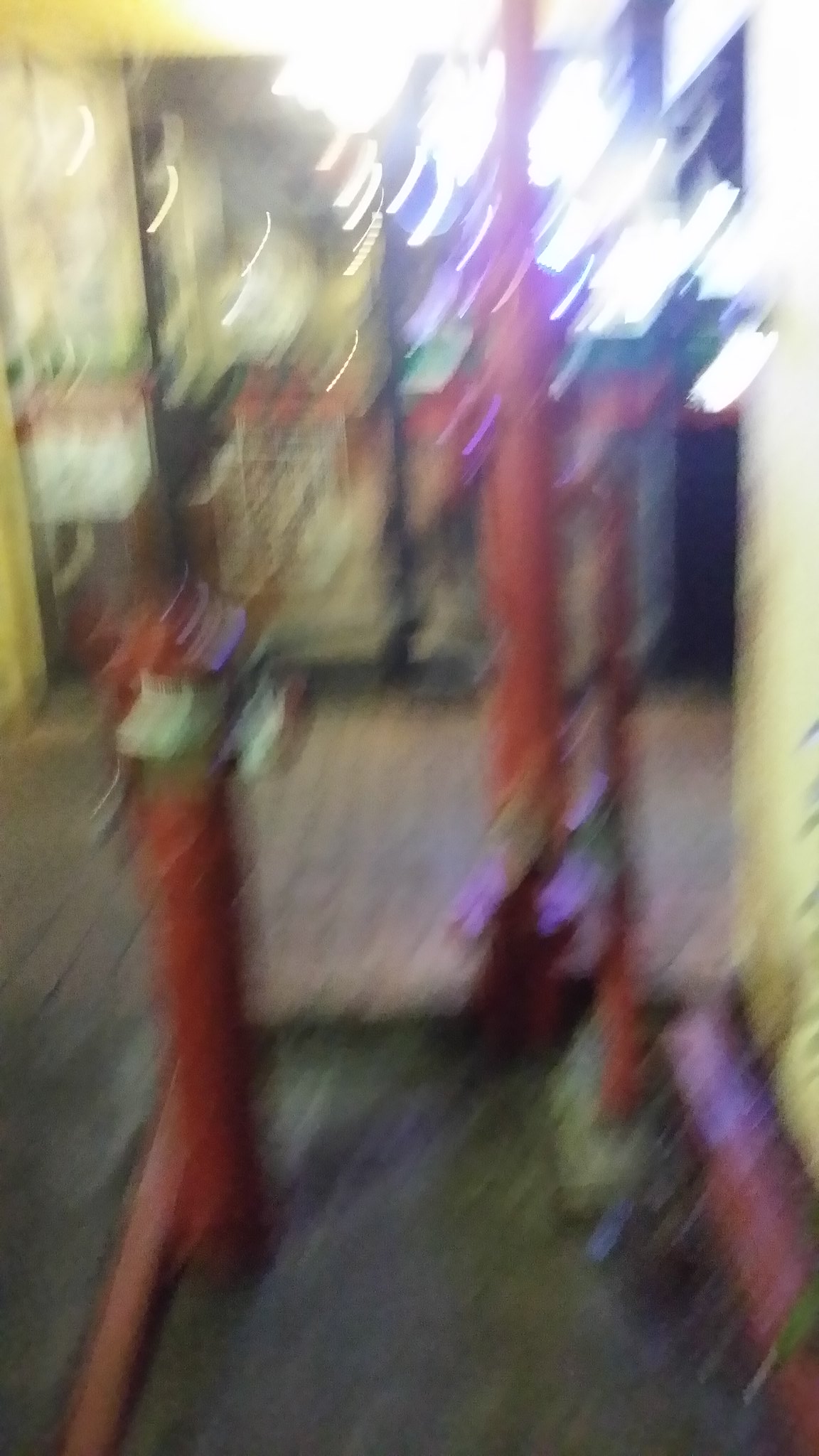This extremely blurry photograph, likely taken in motion with a low-quality camera, depicts a sidewalk in front of a storefront with black-framed glass doors. The floor appears to be made of tan or light reddish hexagon-shaped tiles with dark mortar lines. Positioned near the glass doors are several thin, red, pole-like structures, one of which resembles a fire hydrant. Scattered around the upper right corner of the image are numerous white dots, possibly reflections or lights. Additionally, a warning or danger sign can be vaguely seen on the front door. The overall setting hints at urban or commercial surroundings, with some off-greenish-yellow coloration on the right side, adding to the complexity and confusion of the blurry scene.